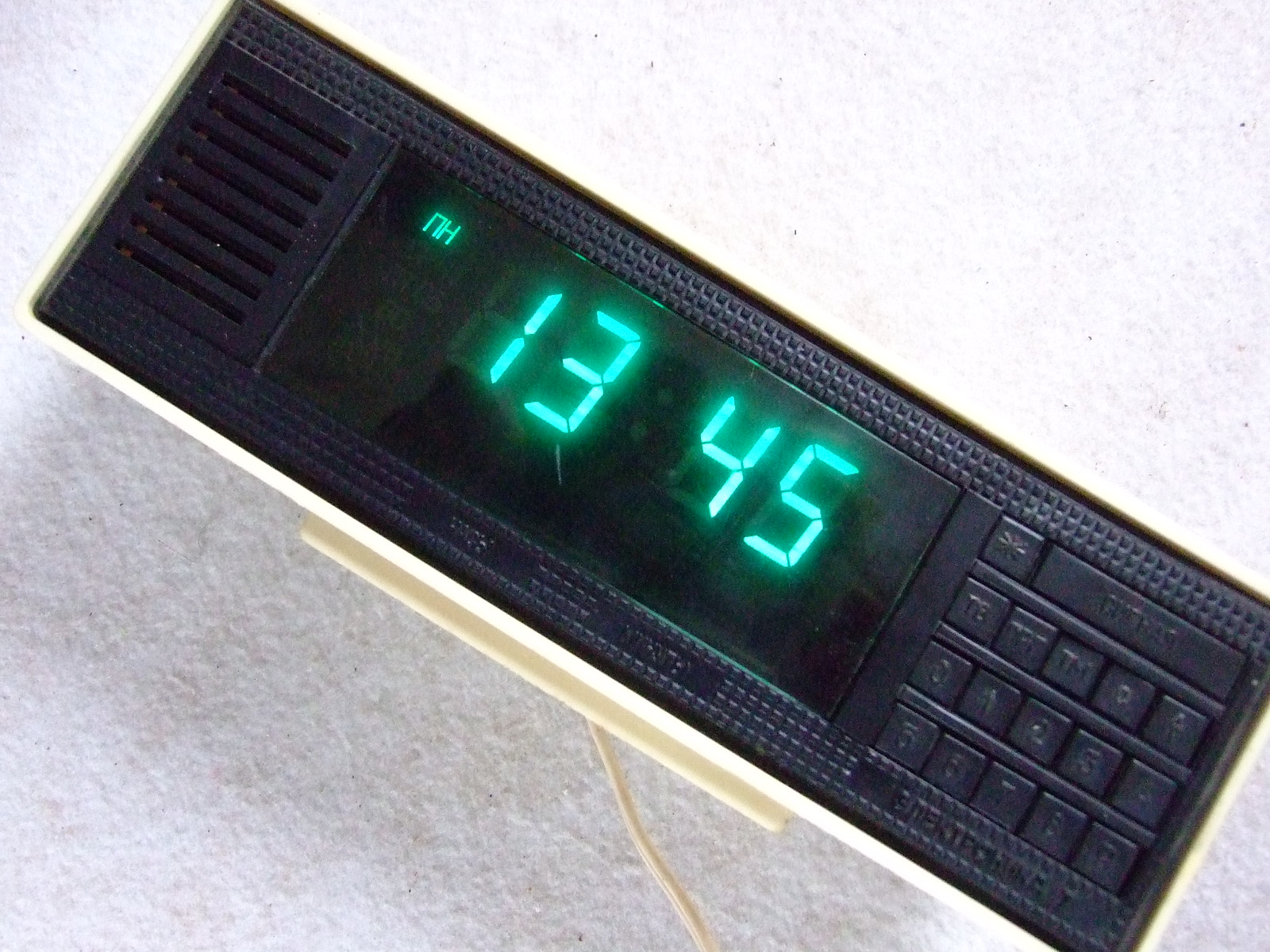The image depicts a rectangular digital clock, positioned diagonally on a white, fuzzy blanket. The base of the clock is white, while its face is black, displaying the time 13:45 in glowing blue LED numbers. On the right side of the clock face, there is a series of small square buttons, and on the left side, there is a speaker made of black plastic. The clock features an 80s or 90s style design. A white cord extends from the bottom of the clock, matching its base. The clock is photographed indoors against a crisp white background.